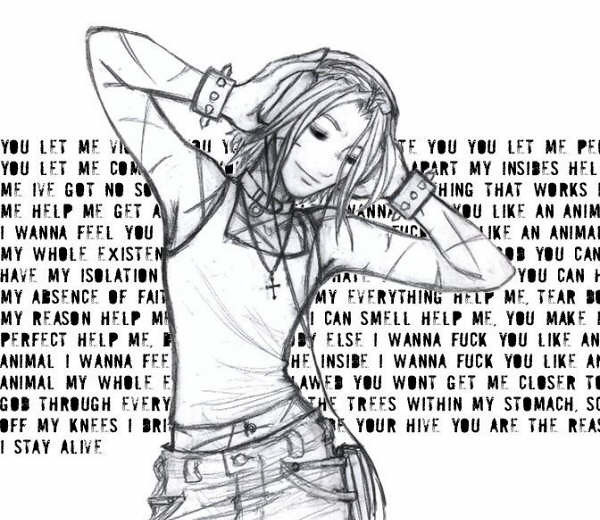This monochromatic, pencil or pen-and-ink sketch portrays a cartoonish or animated teenage girl, likely between 18 and 22 years old, dressed in a light-colored, cropped tank top that reveals her belly button and blue jeans. Around her neck, she's adorned with a cross necklace and a choker, and she sports spiked bracelets on both wrists, evoking a punk rock aesthetic. Her hands, elbows bent, are pressed against her ears as she holds earphones, hinting she's listening to music. Her arms feature X-shaped marks that likely represent self-harm. Behind her, a large paragraph of mostly illegible block-letter text is present, filled with explicit and eclectic phrases, reminiscent of fragmented lyrics or a chaotic manifesto.